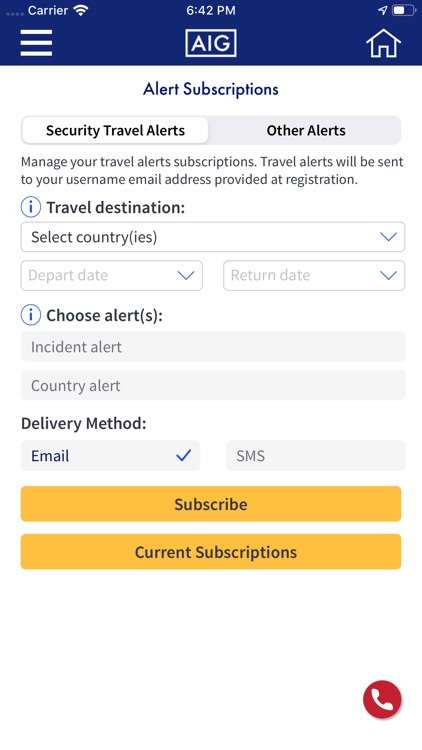On a smartphone screen, the current time reads 6:42 p.m., and the battery is half full. In the top-right corner, the Wi-Fi icon displays three white lines, indicating a strong connection. The screen showcases a travel alert management interface from AIG. At the top, there are symbols for a home, alerts, and subscriptions. Below these icons, there's a section titled "Security Travel Alerts."

The user is prompted to manage their travel alert subscriptions, which will be sent to the email address provided during registration. Options are available to select a travel destination, with a drop-down menu for selecting the country. Additional drop-down menus allow the user to choose departure and return dates. An information icon provides further details about various alert types, including incident and country alerts.

Users can select their preferred delivery method for alerts, with options including email and SMS. A "Subscribe" button is available for confirming current subscriptions. Towards the bottom, a red phone icon implies contact options or emergency assistance.